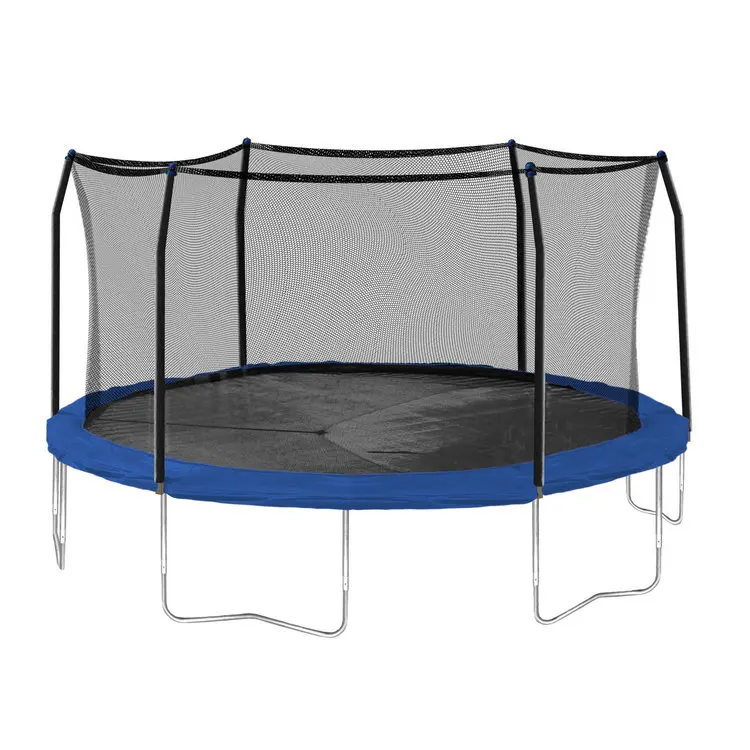This image features a large trampoline with a distinct black jumping surface edged in blue fabric. The trampoline's structure includes six vertical metal poles that support a tall, black mesh netting, forming an enclosure around the jumping area. The netting serves as a safety barrier, likely to prevent users from falling off. This enclosure has a hexagonal shape when viewed from above. The frame of the trampoline itself is silver and square-like, supported by several U-shaped, bent metal pipes that provide stability. The trampoline appears to be photographed against a white background, emphasizing its design and safety features.